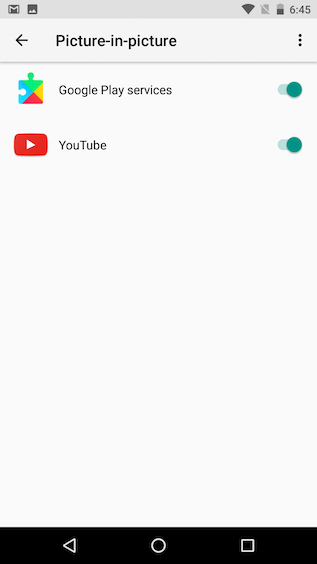This image captures a cell phone screenshot featuring various elements on the screen. At the top, the status bar displays standard cell phone icons such as signal strength, WiFi, and battery level. Below the status bar is the title page, with "Picture-in-Picture" prominently displayed in black font; the initial "P" in "Picture" is capitalized. On the top left, there's a black left arrow (back arrow) indicating navigation options, while on the right are three vertical dots symbolizing additional settings or a menu.

Further down the screen, a section labeled "Google Play Services" is shown with a puzzle piece icon next to it. This service is toggled on, as indicated by the accompanying switch. The last item on the screen is "YouTube," with the recognizable red YouTube icon featuring a white play button at its center, which is also toggled on. The screenshot indicates that the current time is 6:45.